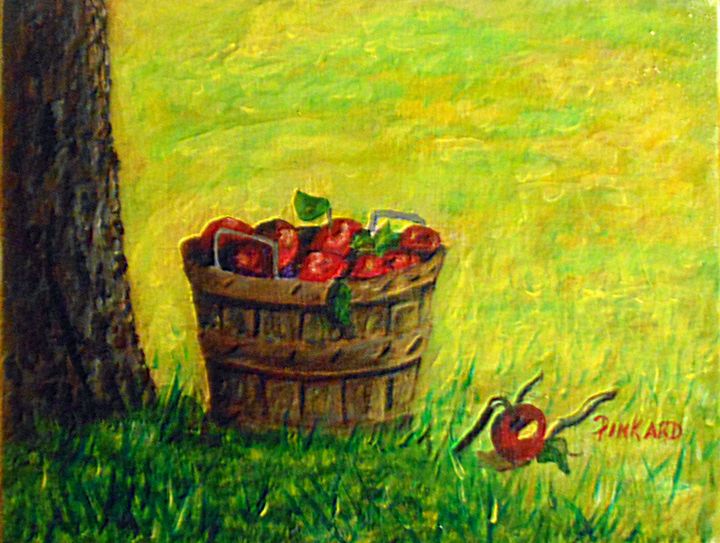This is a detailed oil painting of an orchard scene by the artist Pinkard, whose name appears in red lettering in the right-hand corner. Central to the composition is a rustic wooden basket, constructed from vertical wooden slats held together by a rounded wooden rim and featuring two metal handles. The basket is filled to the brim with apples, likely of the Red Delicious or Gala variety, with their distinct deep red coloration. Some of the apples display the classic green leaves at their tops. One apple has tumbled out of the basket and rests on the grass to the right. The entire scene is set on a lush grassy field, with shades of pink, green, and yellow hues interwoven throughout the grass, creating a vibrant and naturalistic setting. To the left corner of the image, the trunk of an apple tree is partially visible, anchoring the composition and confirming the orchard setting. The background features a meadow with varying greenery, indicating a serene and fertile landscape. The painting captures the tranquility and bounty of the orchard with meticulous detail, from the texture of the wooden basket to the vivid colors of the apples and the nuanced shades of the grass.